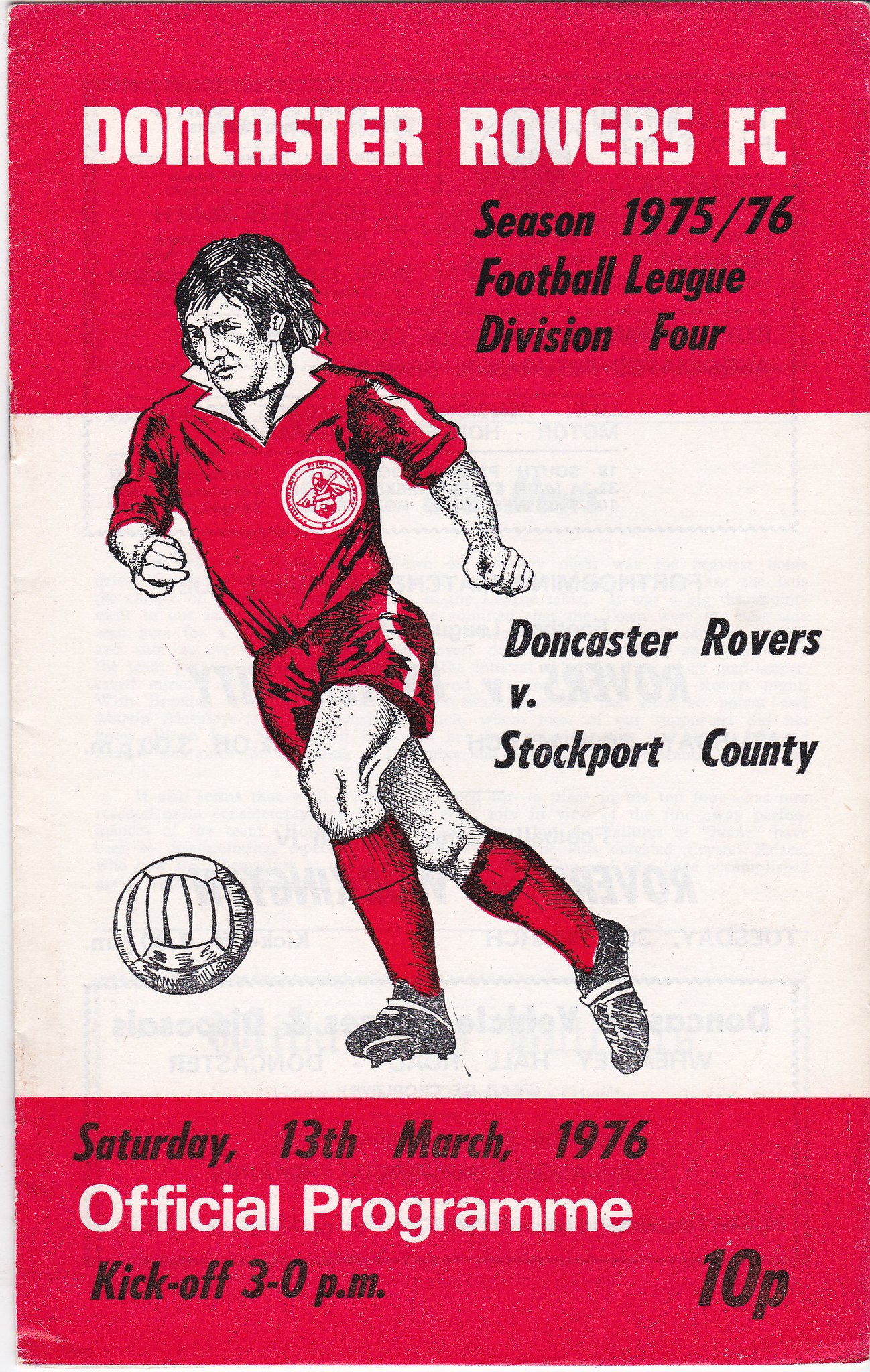This is a detailed drawing featured on the front page of the Doncaster Rovers FC football program from the 1975-76 season in Football League Division 4. The page is divided into three sections with red boxes at the top and bottom and a white or gray band in the middle. At the top, in white text, it reads "Doncaster Rovers FC," followed by "Season 1975-76 Football League Division 4" in black. 

Central to the image is a detailed graphic of a football player, who appears to be an older white man with long hair. He is depicted in mid-action, attempting to kick a white soccer ball. The player is dressed in a red jersey and red shorts with a white stripe down the side, along with red socks and black cleats. His arms are spread out for balance. The player's jersey also features the Doncaster Rovers emblem, which depicts a Viking with a sword and shield, wearing a robe and a helmet with wings.

Across the center band, in black text, it states, "Doncaster Rovers versus Stockport County." Further down, in the bottom red box, the text details the match information: "Saturday, 13th March 1976," followed by "Official Programme" in white, with an extra "e" at the end. Below that, in black text, it reads "Kickoff 3-0 P.M." In the bottom right-hand corner, the price of "10p" is marked in black italics.